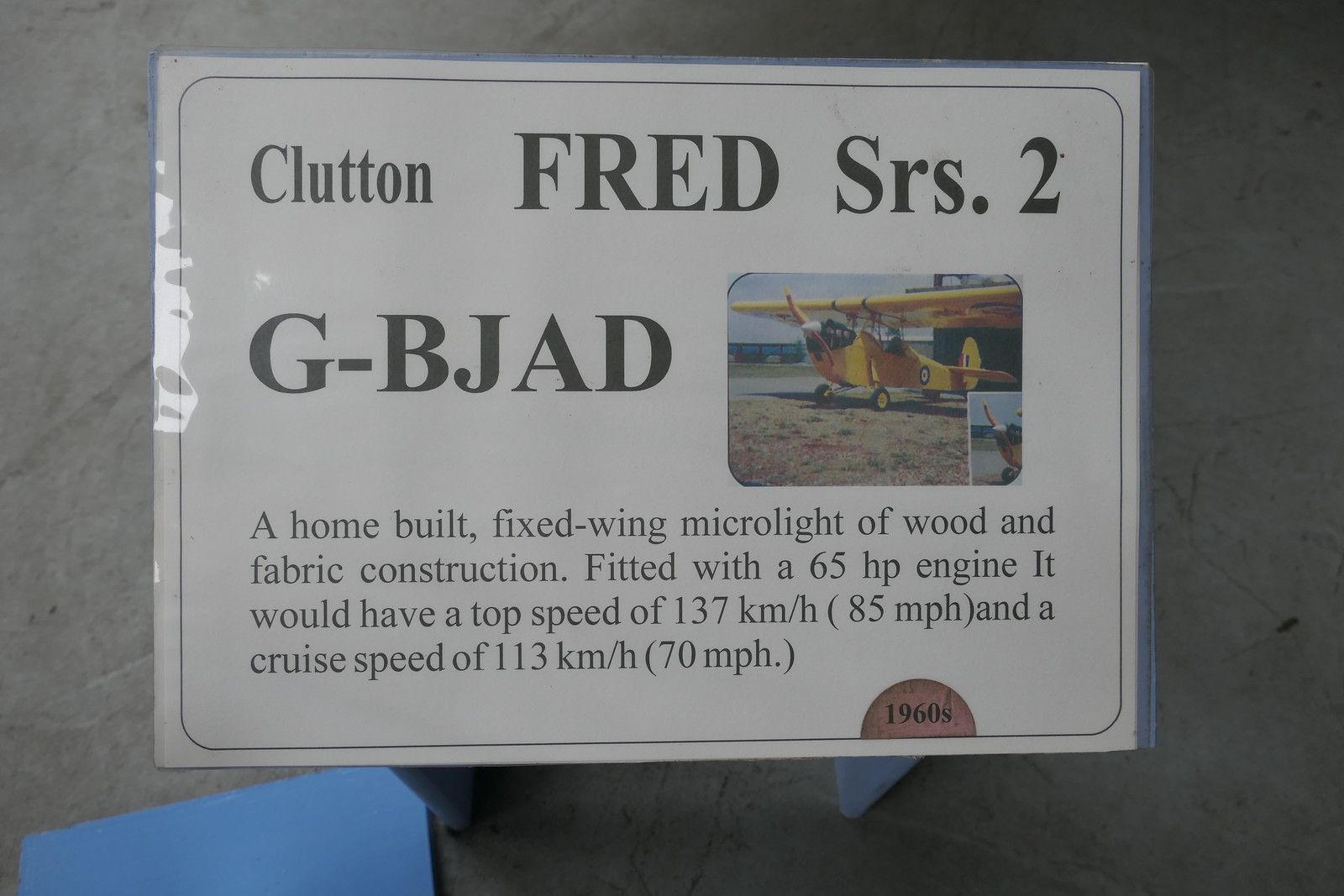This is a laminated, glossy rectangular landscape-shaped signage propped up on a dark, blurred gray background. The poster displays detailed information about an airplane. At the top, in large, bold black letters, it reads "Clutton Fred SRS No. 2" followed by "G-BJAD" beneath it. To the right of the text, there's a small, colorful photograph of a yellow single-engine airplane situated on a beach. Below the photo, the poster further describes the aircraft: "A home-built fixed-wing microlight of wood and fabric construction, fitted with a 65 horsepower engine. It has a top speed of 137 kilometers per hour (85 miles per hour) and a cruise speed of 113 kilometers per hour (70 miles per hour)." The combination of colors on the poster includes black, white, yellow, red, brown, and blue, indicative of the text and the airplane image. The plane is noted to be from the 1960s.